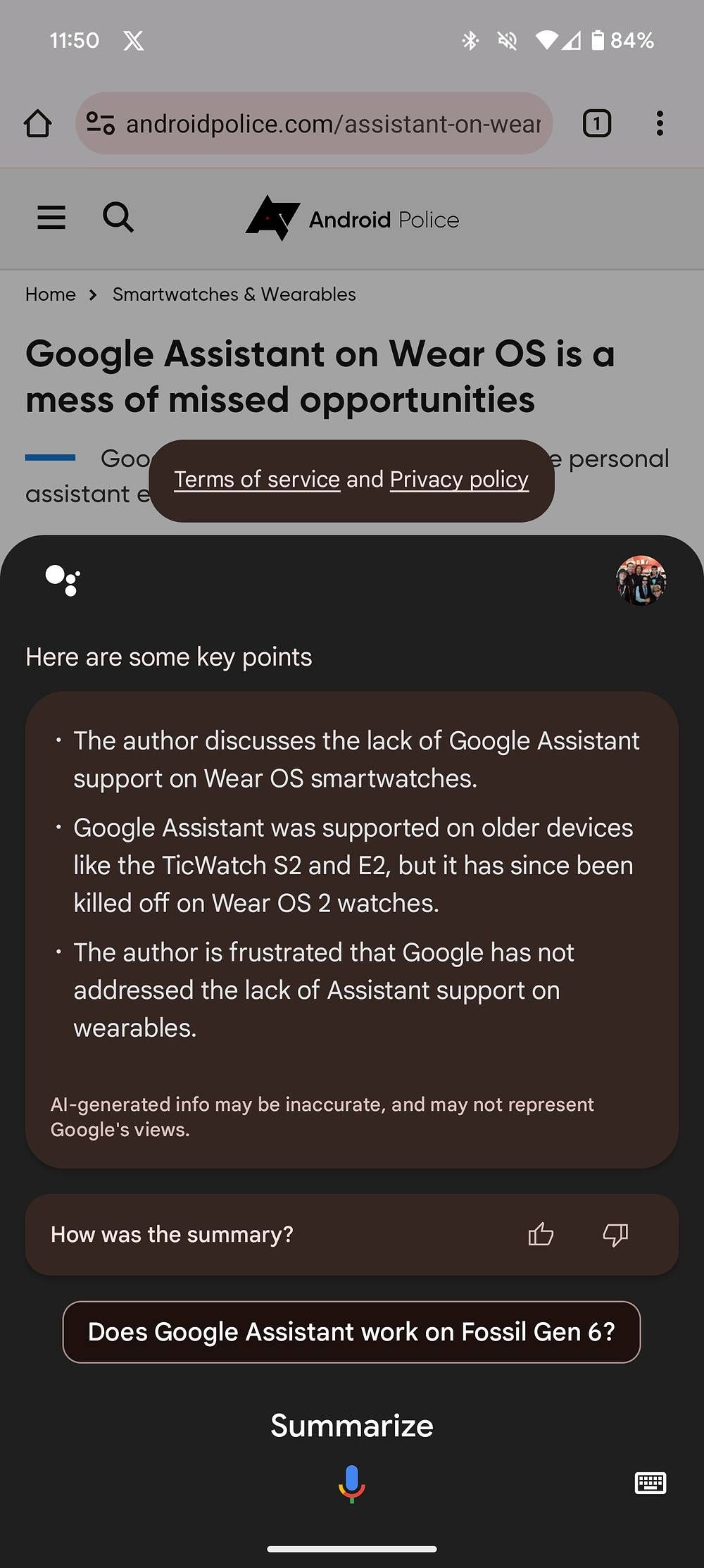This image depicts a screenshot from a mobile device, presented against a gray background. The top half of the screenshot features a status bar with several icons: the time displayed on the upper left as '11:50', and on the upper right, icons indicating Bluetooth connectivity, notifications, Wi-Fi, and cellular signal, along with a battery level of 84%. Directly beneath this status bar is an address bar showing the URL 'androidpolice.com/assistant-on' in black text.

Below the address bar, a search bar for Android Police is visible against a gray backdrop. The main content of the screenshot reveals a headline in large black text, stating "Google Assistant on Wear OS is a mess of missed opportunities." Beneath this headline is a social media post summarizing key points of the article. The post highlights issues discussed by the author, including the inadequate support for Google Assistant on Wear OS smartwatches, despite its previous availability on older devices like the TicWatch S2 and E2.